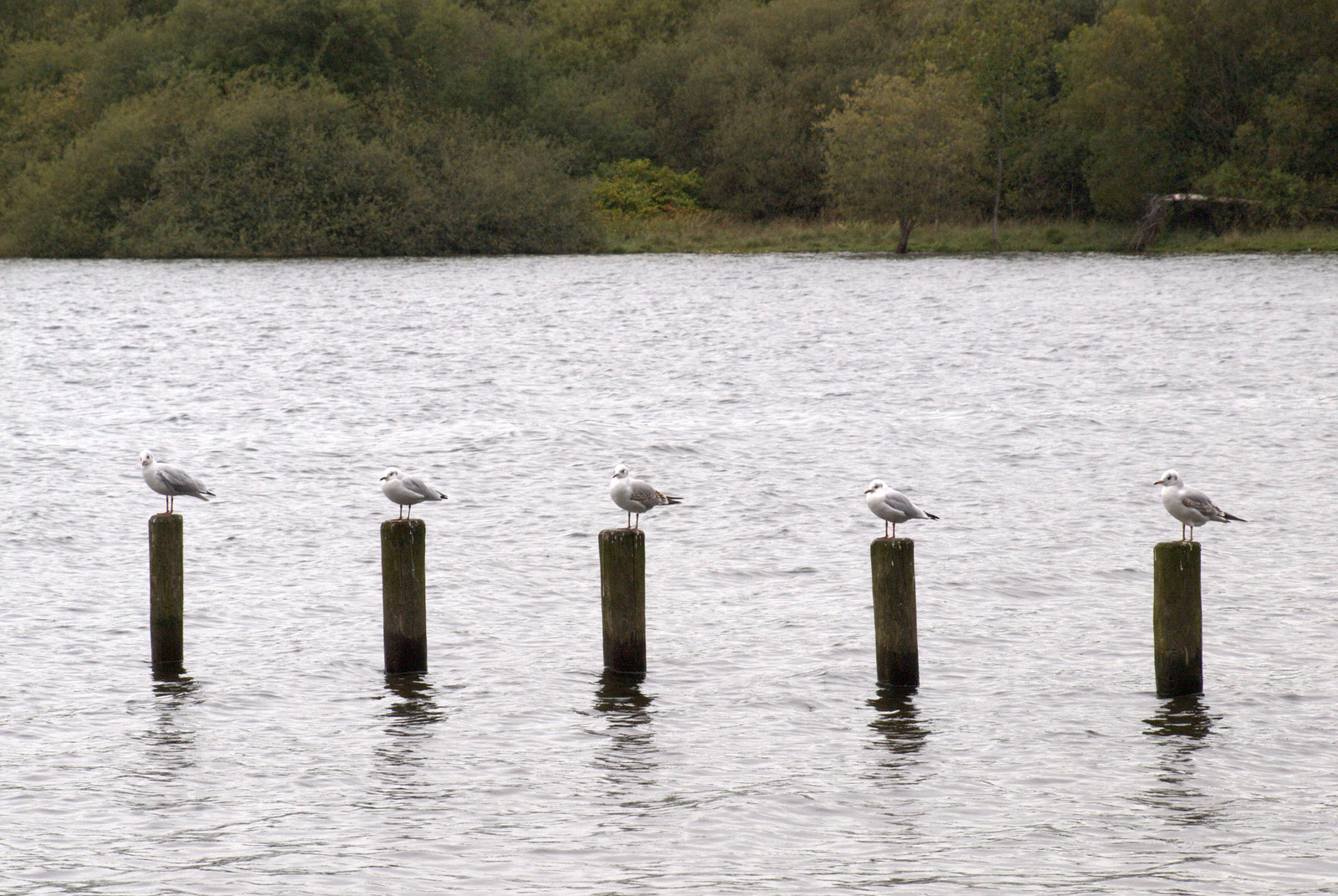In this photograph, we see a serene body of water, either a lake or a river, with slight ripples, giving the water a shiny, gray, and slate-like appearance under what seems to be an overcast sky. Humorously arranged in the bottom third of the frame, five identical wooden posts rise above the water's surface, each topped by a white bird with hints of gray on their wings, resembling pigeons or seagulls. All the birds are perched neatly and uniformly, facing to the left, adding a whimsical touch to the scene. In the top third of the image, the far bank is visible, lined with dense shrubs, grass, and a forest of trees, the greenery showing the slightest touch of seasonal change with tinges of brown and red, suggesting the onset of autumn.